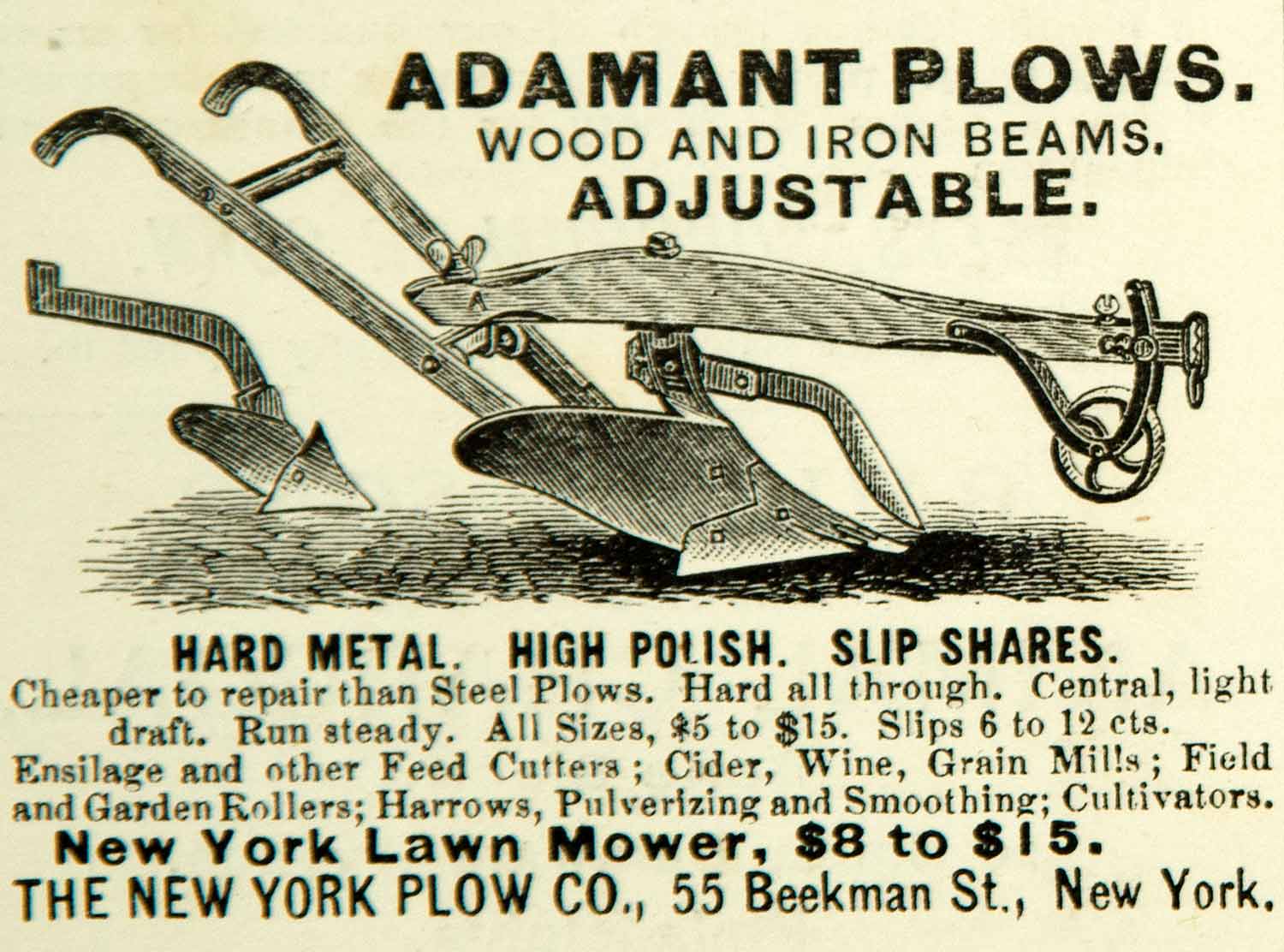The image is an advertisement for a plow tool, presented in a landscape layout with a cream-colored background and black text. At the top, the text reads "Adamant Plows, Wooden Iron Beams Adjustable." A detailed black sketch of the plow, resembling a mechanical contraption with numerous levers and beams, occupies the center. Beneath the sketch, further text highlights the plow's features: "Hard Metal, High Polish, Slip Shares. Cheaper to repair than Steel Plows, Hard All Through, Central Light Draft, Run Steady, All Sizes. $5 to $15. Slips 6 to 12 CTS." Additional text promotes related agricultural tools and machinery, including "Insulage and other Feed Cutters, Cider, Wine, Grain Mills, Field and Garden Rollers, Harrows, Pulverizing, and Smoothing Cultivators," and notes the "New York Lawn Mower, $8 to $15." The advertisement concludes with the manufacturer’s information: "The New York Plow Company, 55 Beekman Street, New York." The entire design features only text and the plow sketch, set against the monochromatic cream background.